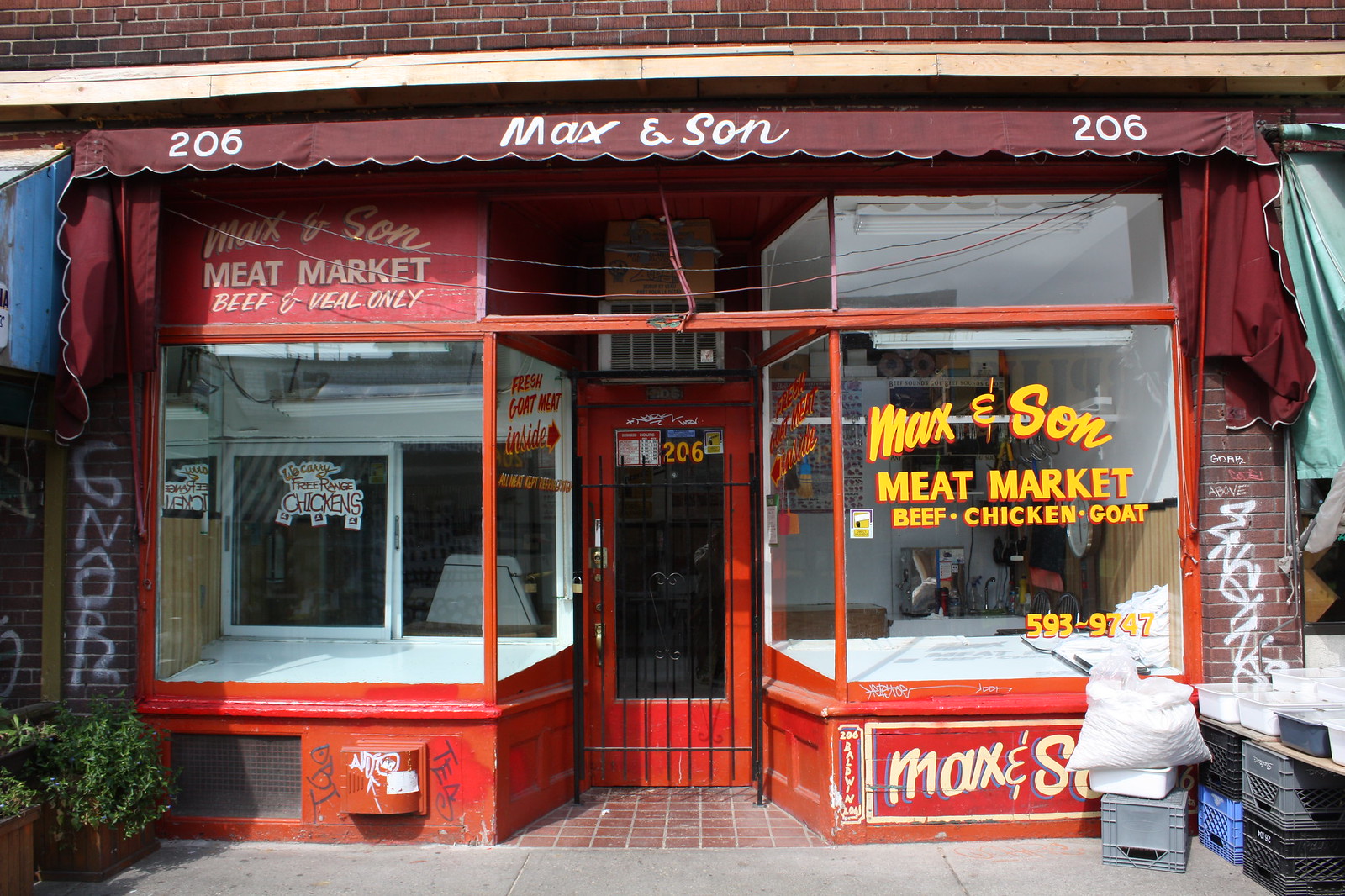The image depicts a storefront of a traditional red brick building that houses "Max and Son Meat Market," located at street number 206. The upper portion of the building includes taller apartments, while the bottom features the meat shop. The shop has a maroon cloth overhang with "Max and Son" written in white.

Below the overhang, the storefront showcases two large square glass windows – one on the left and one on the right. Both display windows are currently empty, suggesting the shop might be closed. The red door in the center has a large see-through glass pane and is reinforced with black metal bars, reminiscent of jail bars, likely for security purposes.

The window on the right bears yellow text advertising "Max and Son Meat Market," specifying they sell beef, chicken, and goat. On the sidewalk in front of the shop, milk crates are stacked with a brown table on top, holding several white plastic containers. Additionally, there are graffiti marks to the left of the shop, and a few small plants are visible in the bottom left corner of the image. The phone number provided on the display is 593-9747.